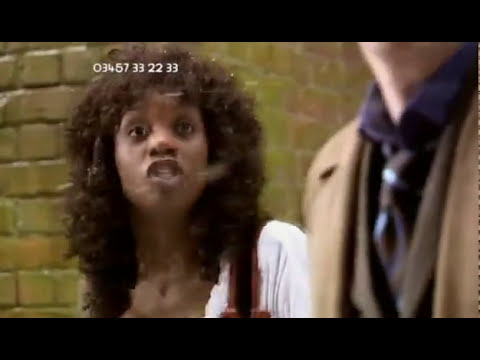The image is a somewhat blurry screenshot from a video, depicting two individuals against a greenish brick wall backdrop. On the left, an African-American woman with long, curly hair cascading to her armpits is seemingly in mid-conversation. Her mouth is partially open, revealing her teeth. She is adorned in a white shirt with a bag strap over her left shoulder, and she appears to be wearing a necklace. Floating above her hair are the white numbers "0345 733 2233," indicative of a screen grab from a video. To the right, a blurred partial view of what appears to be a man is visible from below the chin to the chest. He is dressed in a light brown suit jacket over a brown vest, a blue shirt, and a dark brown tie with white or blue stripes. The woman is looking towards the man, engaging in dialogue.